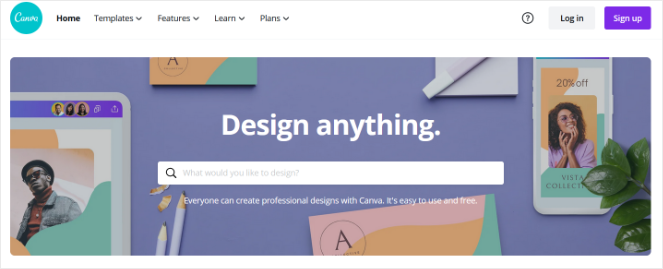A detailed photographic screenshot of a webpage primarily adorned in white, with accents of blue, black, purple, green, pink, orange, and light green hues. In the upper left-hand corner, there is a blue circle featuring the word "Canva" in white lettering. The navigation bar at the top contains several tabs, including "Home," which is selected and highlighted in bold black font. Additional tabs include "Templates" with a dropdown menu, "Features" with a dropdown, "Learn" with a dropdown, and "Plans" with a dropdown.

Adjacent to the navigation bar, there is a circular icon with a question mark. Next to it, a gray login button with black text is positioned beside a purple signup button displaying white text. Below this navigation area, a prominent purple banner spans the width of the page, displaying the white, bolded text "Design anything" at its center.

Beneath the banner, a search bar stands out with the placeholder text, "What would you like to design?" Near the search bar, there is an image depicting two pencils accompanied by pencil shavings. The text alongside the image states, "Everyone can create professional designs with Canva. It's easy to use and free." Additionally, visuals of a tablet and a mobile device are presented, underscoring the platform's accessibility across different devices.